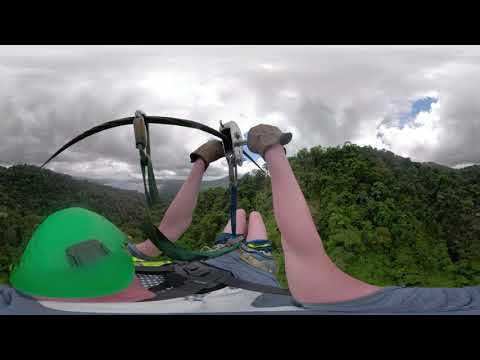The photograph is a full-color, horizontally rectangular image taken outdoors on an overcast day, framed by black borders at the top and bottom. The scene captures a thrilling moment where you, a likely Caucasian male wearing a green helmet, brown gloves, and a gray T-shirt with shorts, are ziplining over a lush, tree-covered mountainous landscape. The image, possibly taken with a helmet cam, exhibits a fish-eye lens effect, creating a distorted and rounded appearance. The ziplining setup includes a handlebar to which you are clinging, and you are secured by a harness with blue strapping. Your legs are extended, emphasizing the suspended, mid-air exhilaration of the activity. The background features low mountains dense with green foliage, spanning bushes, shrubbery, and tall trees. Above, the sky is dominated by grey and white clouds, with a small patch of blue visible in the top right corner, conveying a sense of looming weather.